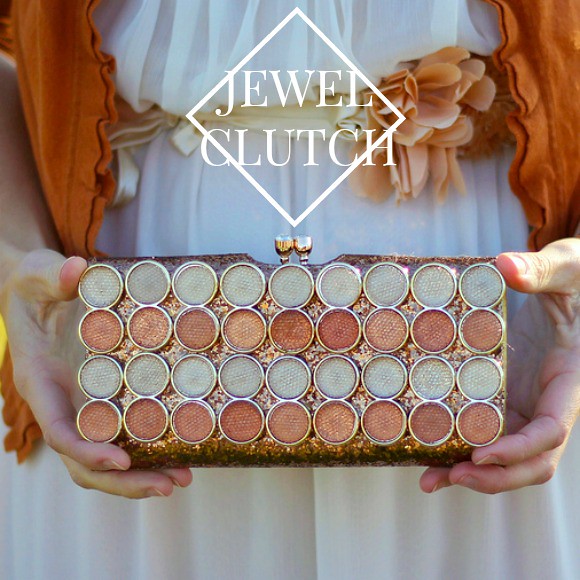In the image, a woman is shown from the chest down, wearing a white dress with a cloth belt featuring a red flower. An orange vest or cardigan, with short sleeves, overlays her dress. She is holding a tray or clutch, which contains four rows of small circular containers, totalling 36 in all. The top and third rows consist of white circles, while the second and bottom rows include shades of red, pink, peach, and blush. Above the clutch, in white text within a white diamond outline, the words "Jewel Clutch" are prominently displayed. The clutch has a metallic sheen, displaying hues of orange and gold. The woman's hands are the focal point as she presents the clutch, emphasizing the detailed organization and color variation within the item.